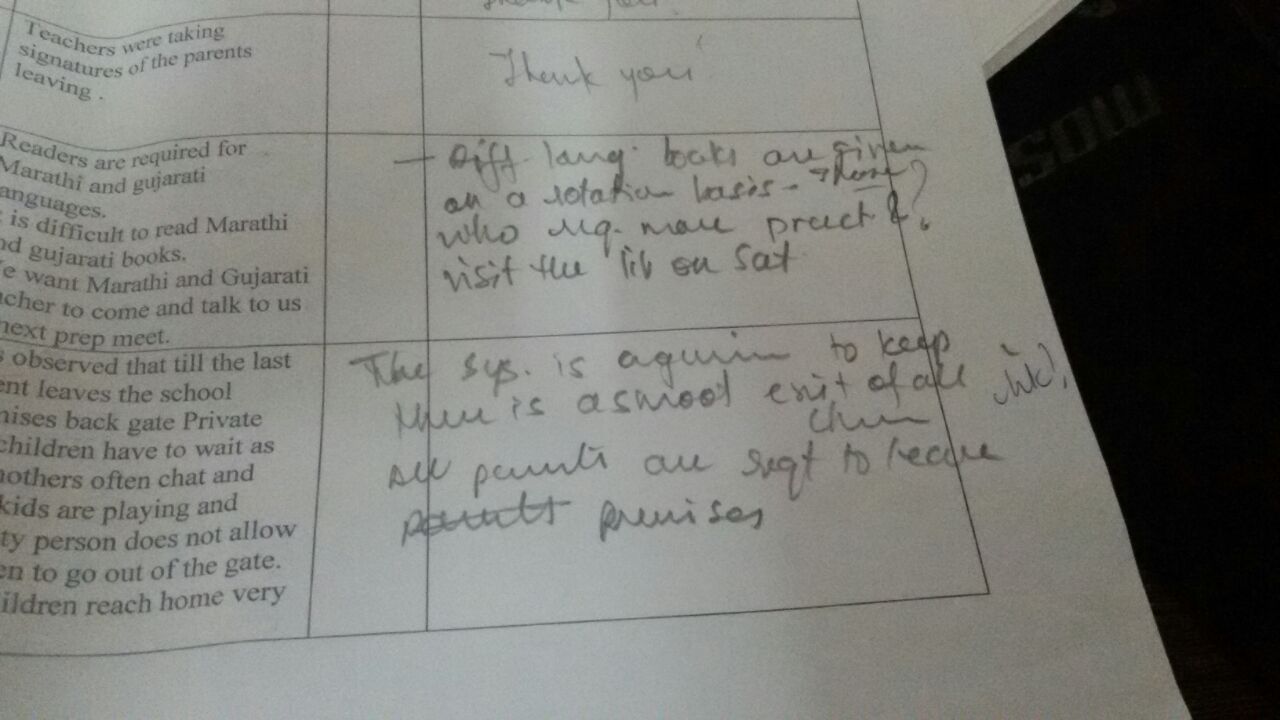This photograph showcases a printed document on a white piece of paper, presumably from a school library, with typewritten text on the left and handwritten notes in pencil on the right. The left side features structured information in black ink, while the right side contains several handwritten annotations, some of which are partially legible.

At the top left corner, the typewritten text reads, "teachers were taking signatures of the parents leaving," with the adjacent handwritten note simply stating, "thank you." Further down on the left, another printed note specifies, "readers are required for Marathi and Gujarati languages. It is difficult to read Marathi and Gujarati books. We want Marathi and Gujarati to come and talk to us next prep meet." The corresponding handwritten section here is largely illegible, although it partially reads, "different language books are given on a relative, on a relation basis."

Towards the bottom, the printed text mentions, "observe that until the last leaves the school, private children have to wait as others often chat and kids are playing," but the adjacent handwritten annotation is fragmented and challenging to decipher, with phrases like, "this system is a choir to keep," and "school exit at all." The bottom box is cut off, making both the printed text and handwritten notes therein difficult, if not impossible, to read.

Overall, the document appears to list requirements and observations related to linguistic needs and school processes, supplemented by fragmented handwritten notes that add a personal or situational context, yet are hard to fully decipher.